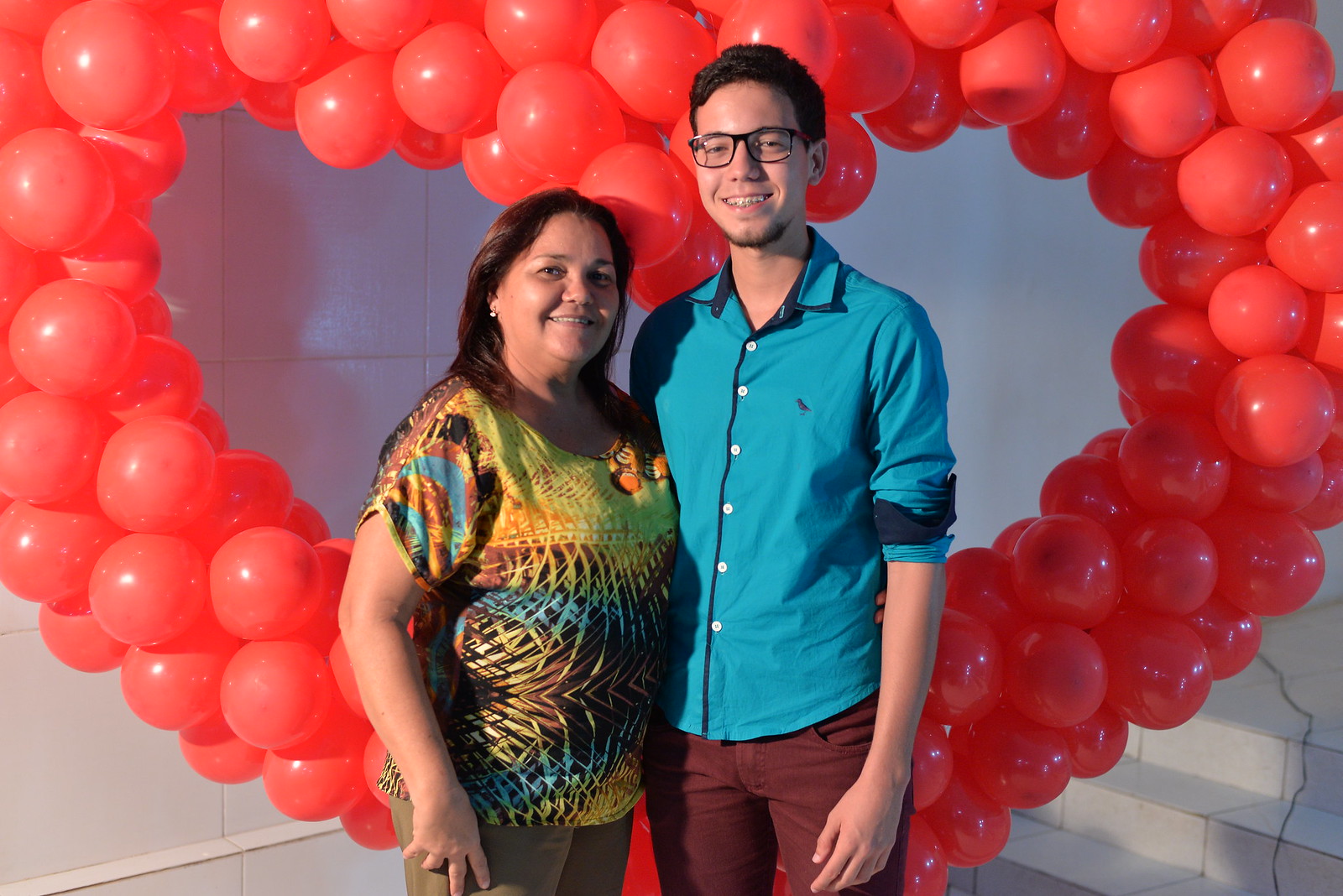In this photograph, a mother and her son are posing happily in front of a heart-shaped balloon arch, likely set up for a Valentine's Day event, a prom, or a homecoming dance. The balloon sculpture behind them is made of bright red and pinkish balloons, forming a large, eye-catching heart. The mother, who appears to be in her forties, stands on the left wearing a vibrant shirt featuring yellows, greens, browns, and blues, paired with tan pants. She is shorter and has a round face with chubby cheeks. Next to her is her son, a young man in his late teens or early twenties, wearing a bright blue button-down shirt with rolled-up sleeves and burgundy pants. He has dark hair, glasses, and a small goatee on the bottom of his chin. They both look cheerful and content as they smile for the camera, suggesting a close family bond rather than a romantic relationship.